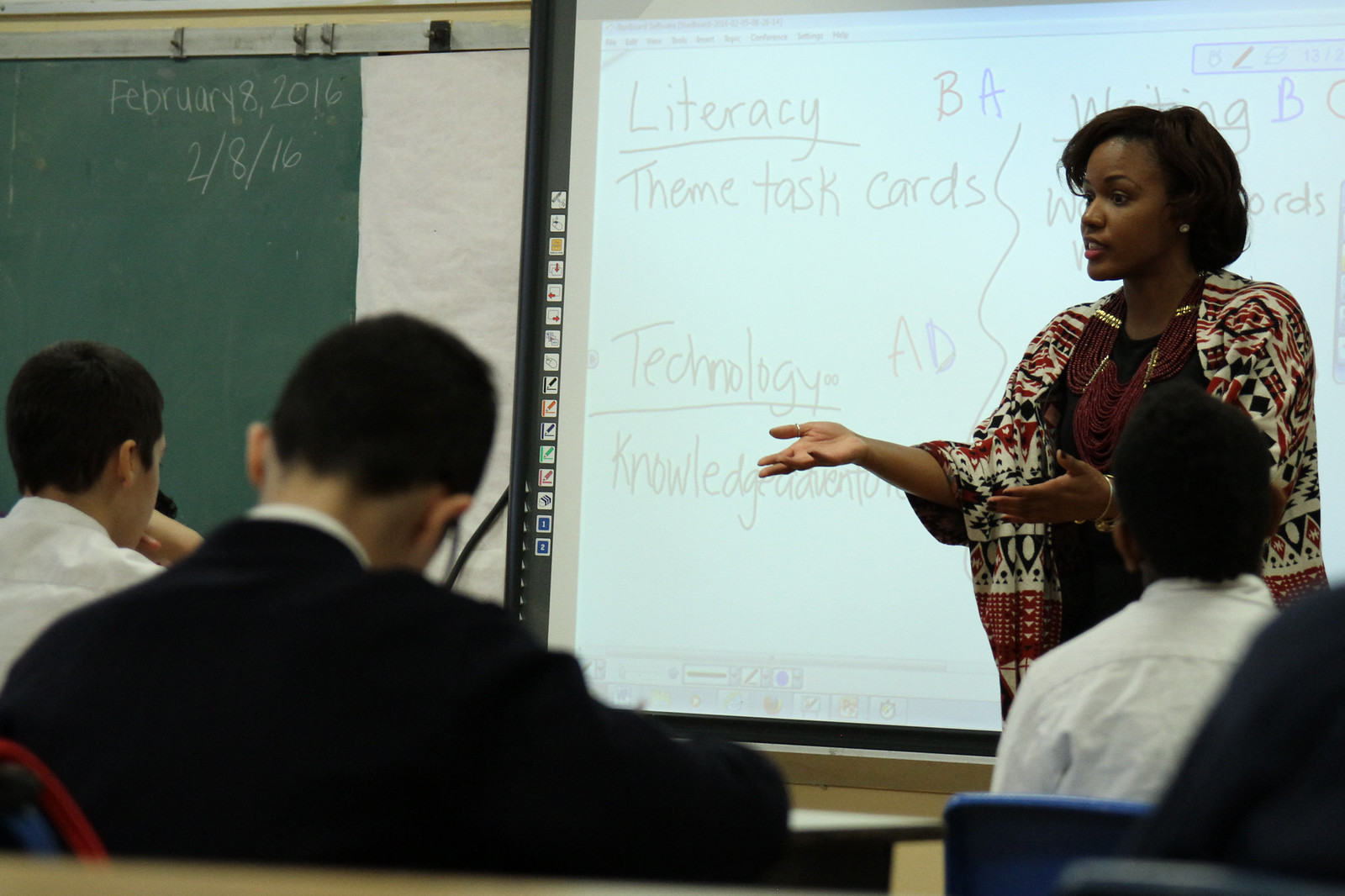The image depicts a detailed classroom scenario, likely a college or high school setting, with a central focus on a black woman who appears to be the teacher or professor. She stands prominently in front of the class, her arms outstretched as she lectures, emphasizing her points. She is stylishly dressed in a shawl with a red, white, and black tribal pattern over a black dress, adorned with a beaded ruby and gold necklace. Her short hair and animated posture mark her engagement with the students, who are seated at their desks.

To the left of the teacher is a green chalkboard with white writing, including the date "February 8, 2016." To the right is a projection screen displaying words such as "Literacy, B.A.," "Theme Task Cards," "Technology, A.D.," "Knowledge," and potentially "Writing, B.C.," partially obscured by her. In the foreground, three male students with short dark hair are visible; one in a white shirt on the far left, one in a black shirt closer to the camera, and another in a white shirt on the far right, all facing away from the camera and focused on their desks. The overall scene portrays an engaging educational environment with an emphasis on literacy and technology.